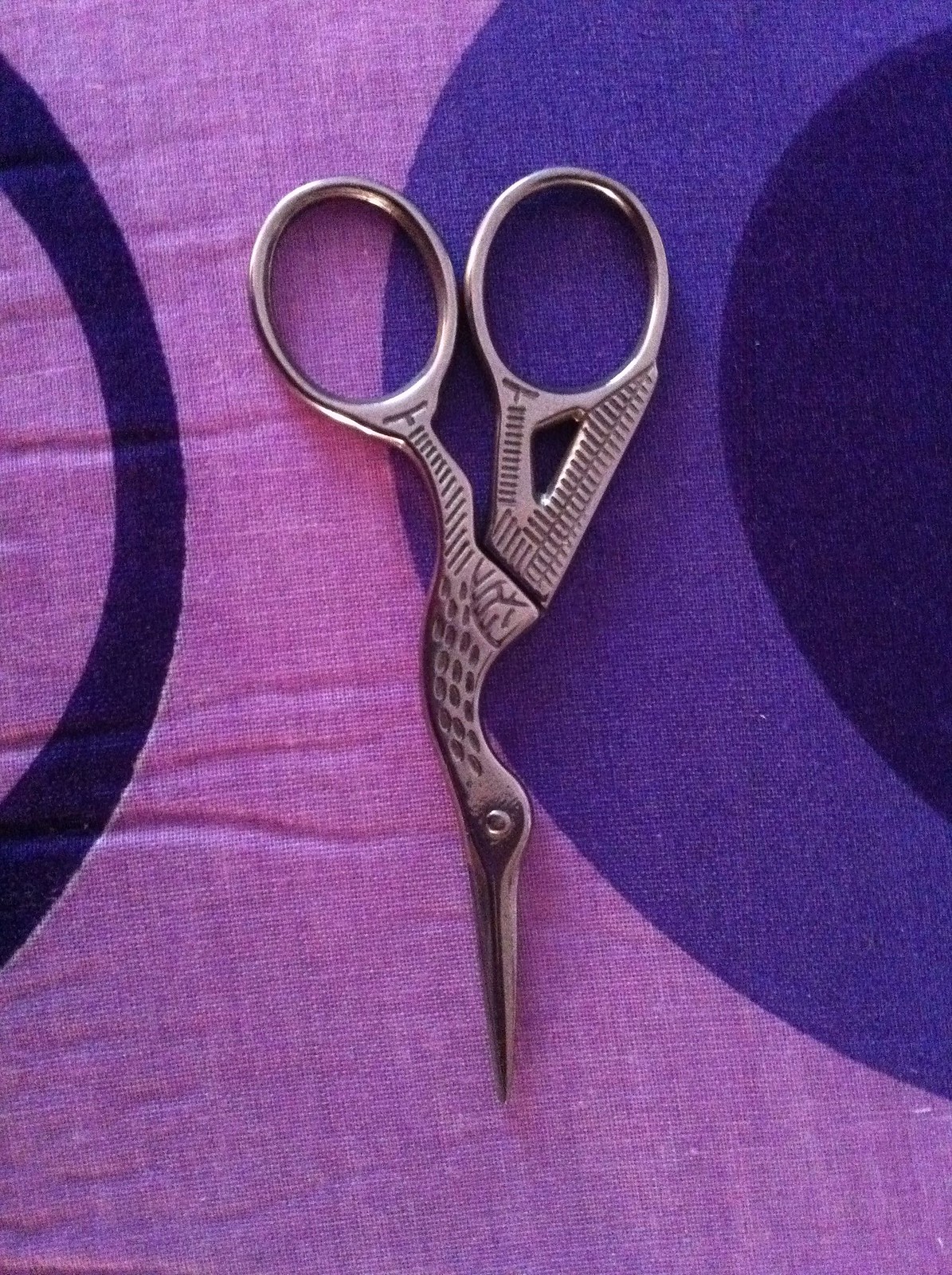This is a detailed, up-close photograph of a pair of classic, small, silver sewing scissors designed to resemble a bird, possibly a goose or a similar bird in flight. The bird motif is intricately rendered, featuring etched feathers and an eye. The cutting blades form the bird's beak, and the finger holes mimic the bird's feet. The scissors are positioned nose-down, resting on a vibrant, multi-toned piece of fabric. The fabric showcases a rich gradient of colors from dark purple to pink-violet, adorned with distinct patterns: a black stripe on the left, a large blue circular stripe in the center with a black semi-circle at the top right edge. The overall impression is that of a well-maintained, delicately crafted tool lying on a striking, colorful fabric, offering a rich visual composition.